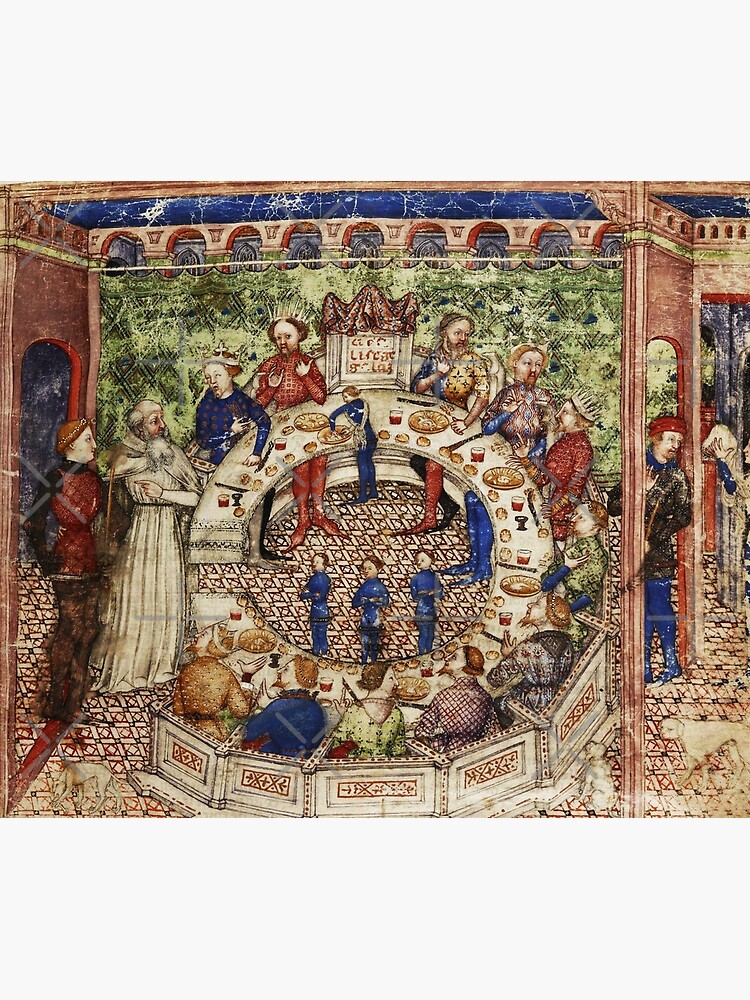This image depicts a detailed and colorful medieval painting, potentially a mural, showcasing a scene from centuries ago. At the center, there is a circular table surrounded by 13 figures clad in various outfits: blue, red, gold, green, and checkered patterns. Notably, figures on the upper left and right sides of the table wear crowns, suggesting royalty. There are four small figures in blue outfits, possibly servants, standing within the inner circle of the table. 

The backdrop of the scene includes a blue-tinted ceiling adorned with brown arches above the table. The floor is tiled and patterned, enhancing the scene's intricate details. On the left side, there is a doorway, while another doorway on the right side shows a person standing and gesturing towards another figure who is nearly out of the frame. The area around the table showcases a green, grass-like background, complementing the overall setting. The depiction of the people and the architectural elements suggests a seminar or a meal taking place, reflective of a historical period long past.